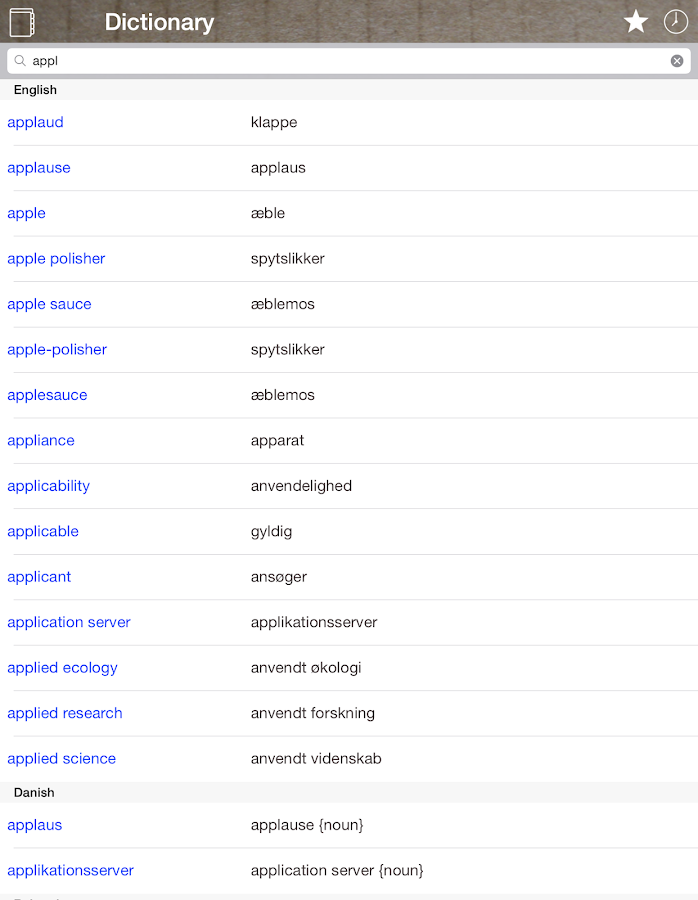This image is a screenshot of a dictionary app displayed on a smartphone. In the upper left corner, there is a small thumbnail of a book. Across the top of the screen, the word "Dictionary" is prominently displayed. Adjacent to this title, there are three icons: a star representing 'favorites,' a clock probably indicating 'recent searches' or 'history,' and another icon whose function is not clearly specified.

The main interface shows a search bar with the letters "APPL" entered into it, and a small 'x' button on the right side of this bar allows users to clear the search field. Below the search bar, the word "English" indicates the language currently being searched.

The search results for "APPL" are listed below, starting with "Applaud," defined briefly as "Clap," followed by the noun "Applause." Next on the list is "Apple," phonetically spelled "A-E-B-L-E," and "Apple Polisher," translated as "Spike Slickter." The term "Applesauce" is shown twice, corresponding phonetically to "Abel Moss." The word "Appliance" appears, phonetically spelled "App-ar-ott."

Other entries include:
- "Applicability," phonetically "Av-en-ven-del-ig-ted."
- "Applicable," rendered as "Glig-lig."
- "Applicant," recorded as "An-sog-er."
- "Application Server," with a straightforward phonetic spelling.
- "Applied Ecology," noted as "Av-ent-o-col-og-y."
- "Applied Research," phonetically "Av-ent-or-ski-nning-oo."
- "Applied Science," indicated as "Av-ent-vi-den-skab-danish."

Following these entries, the word "Applause" is repeated, described twice as a noun. Lastly, "Applicant-so-sa-ser-ver" and "Application Server" appear again, both labeled as nouns.